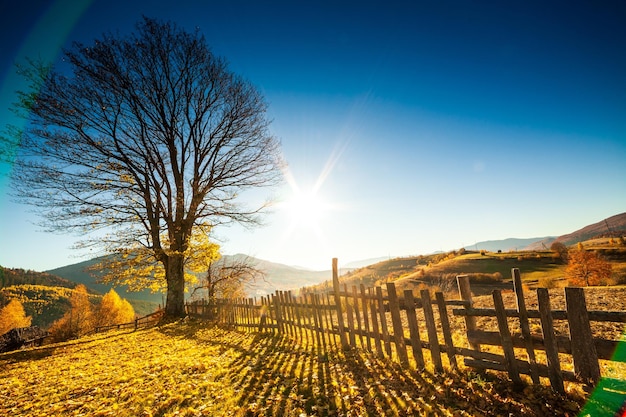This stunning outdoor photograph captures a clear, deep blue sky that transitions beautifully from dark to light towards the horizon. Although the sun itself isn't visible, its white rays stretch majestically upwards, adding a sense of luminescence to the scene. In the background, majestic mountains and rolling hills frame the picture. The sunlight bathes a field in a warm lime-green hue, highlighting the autumn foliage. On the right side of the image stands an old, leaning wooden picket fence, casting intricate shadows on the lush green grass below. The scene is dotted with yellow leaves, some still clinging to a windswept tree with bare black branches, emphasizing the approach of winter. The vibrant colors and serene composition evoke a feeling of tranquility and natural beauty, making it an excellent example of high-quality photography.